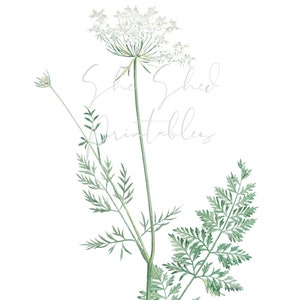This artistic drawing prominently features a detailed depiction of a Queen Anne's lace plant set against a white background. At the center of the image is the primary flower with a long, light green stem, characterized by intricate, delicate detailing that highlights its fine structure and complex beauty. Flanking the central flower, there are two fern-like leaves—one on each side—with the left leaf appearing sparser compared to the right. Additionally, a smaller flower with its own thin stem is positioned nearby. The entire scene is subtly framed at the top by faint white lettering that appears to read "She Shed Printables," although the text is so lightly inscribed that it is barely legible. The drawing is minimalist in composition yet rich in detail, offering a nuanced and finely crafted representation of the plant. The lower portion of the image is cropped just enough to leave a few leaves visible at the edges.